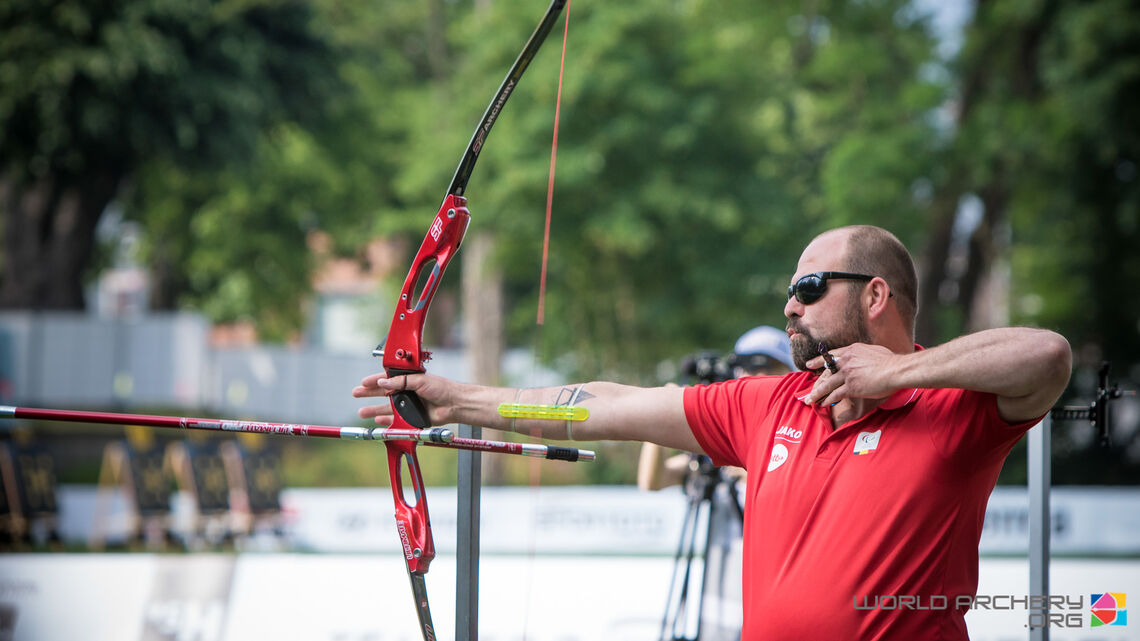In this horizontally aligned rectangular image, a man with a shaved head on top and brown hair on the sides and back is pulling back the string to shoot an arrow from a black and red bow. He has a neatly trimmed brown mustache and beard and wears black sunglasses. Dressed in a red polo shirt, he is positioned on the right side of the image, facing left. His left arm is pulled back with his hand under his chin, as he prepares to release the red and silver arrow. His right hand grips the bow, and the freshly released arrow is visible, streaking towards the left. The blurred background features tall trees and a snippet of blue sky in the upper right corner. Additionally, a man holding a camera can be seen slightly to the left behind him. At the bottom right of the image, "WORLDARCHERY.ORG" is printed in gray all-caps, accompanied by a small, colorful square logo.